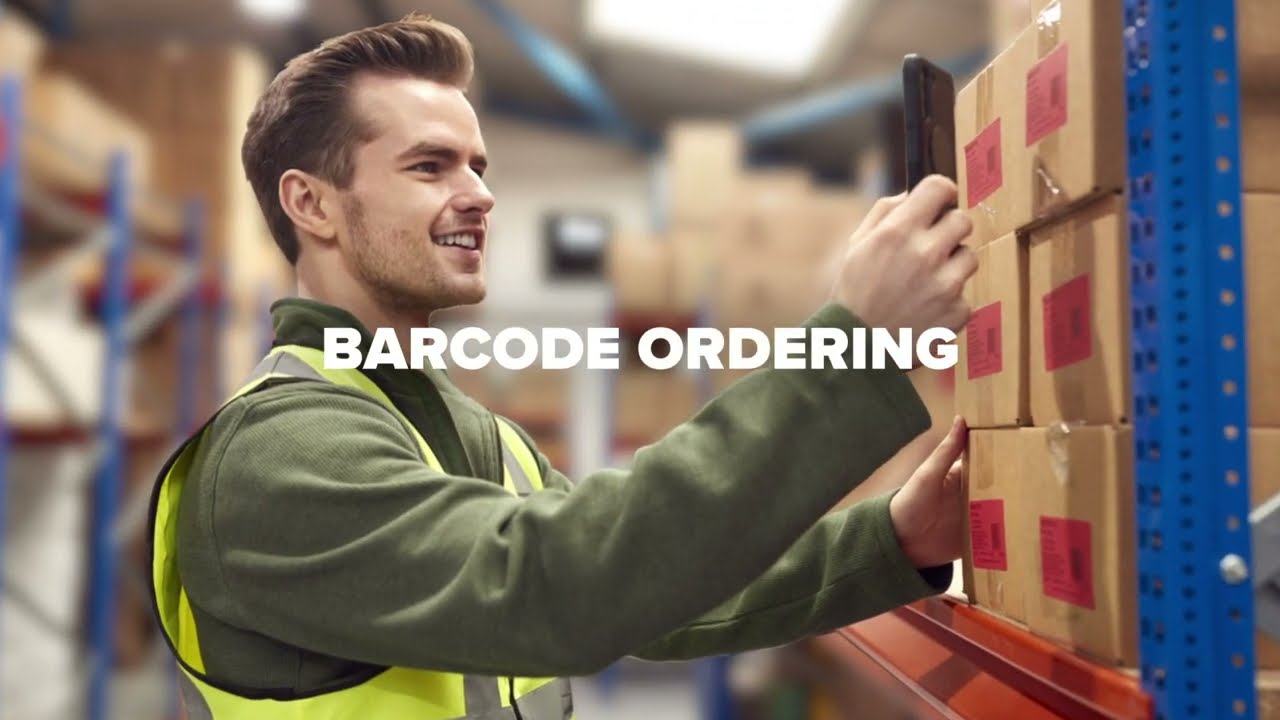The image captures a logistics-focused scene within a warehouse setting. At the forefront stands a white male employee with slightly balding, blonde-brown hair and a smiling expression. He is dressed in a green long-sleeve shirt and a neon yellow safety vest, identifiable by some as a neon green hue. The man is engaged in scanning barcodes using his cell phone on a stack of six brown cardboard boxes with red labels. These boxes are situated to his right, behind a bright blue vertical pole and on orange-painted shelves supported by blue framing and plain silver support braces. The background of the image shows the expansive warehouse space with rows of similar shelves and stacks of boxes, creating a busy yet orderly environment. Amidst this scene, white text in the center of the photo reads "barcode ordering," highlighting the task being performed.